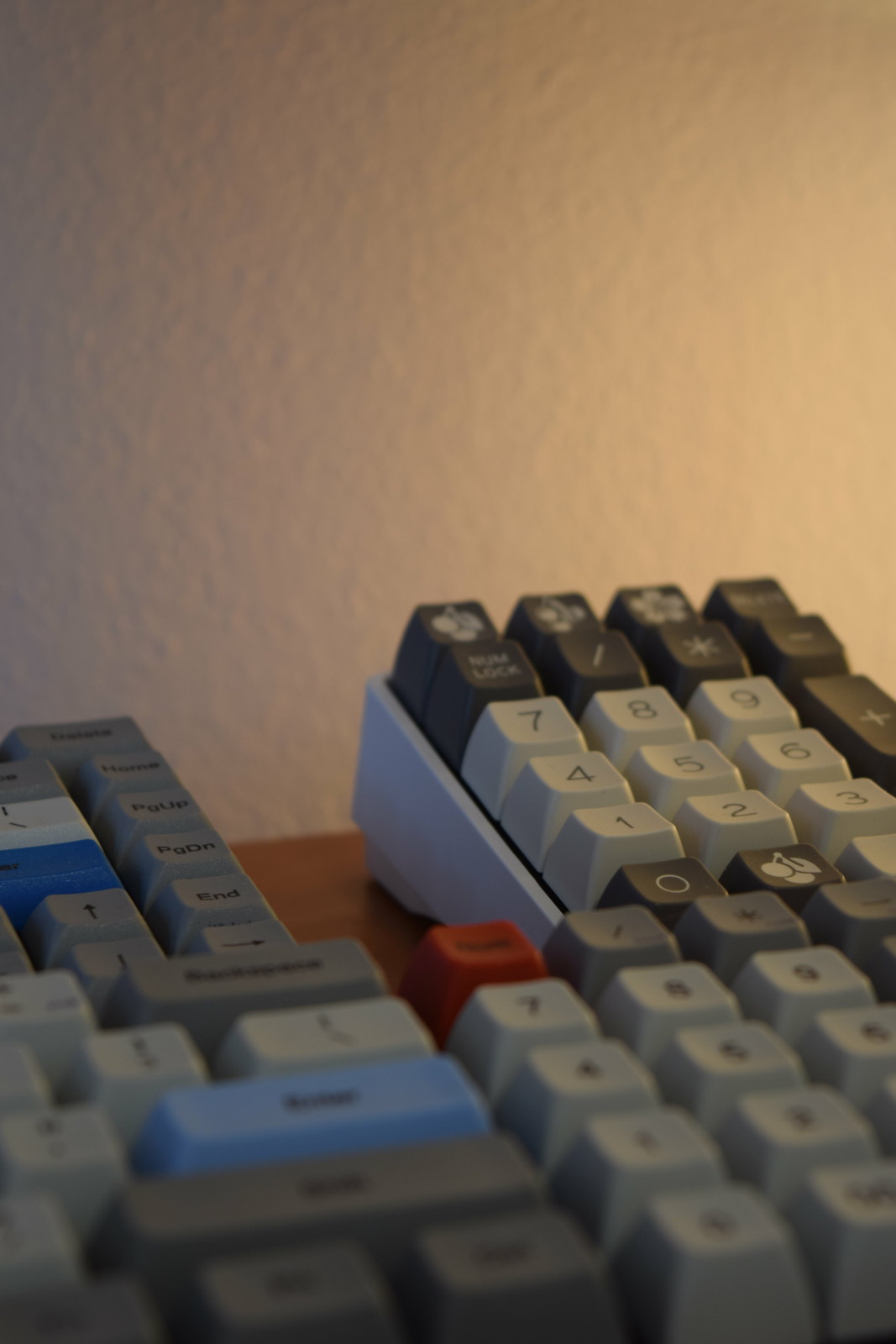The photograph is a close-up of several old-fashioned mechanical keyboards, seemingly pushed together on a dark reddish-brown wooden table. The scene is lit poorly, possibly illuminated only by a desk lamp, casting a peculiar light on the arrangement. Against a patterned white wall, the keyboards exhibit large, chunky black keys with mostly grey caps, apart from sporadic colorful keys.

In the foreground, some keys, like backspace, enter, and shift, stand out, with backspace and shift in grey and enter in blue. Further back, a number pad with the red "num lock" key captures the focus. Additional detail includes two random cherry keys and one sakura key, adding a touch of oddity. The keyboards are positioned in such a way that the image requires a head tilt to the left, providing a tilt-shift visual effect. Key elements like page-up, page-down, and various numeric keys highlight this distinctive setup.